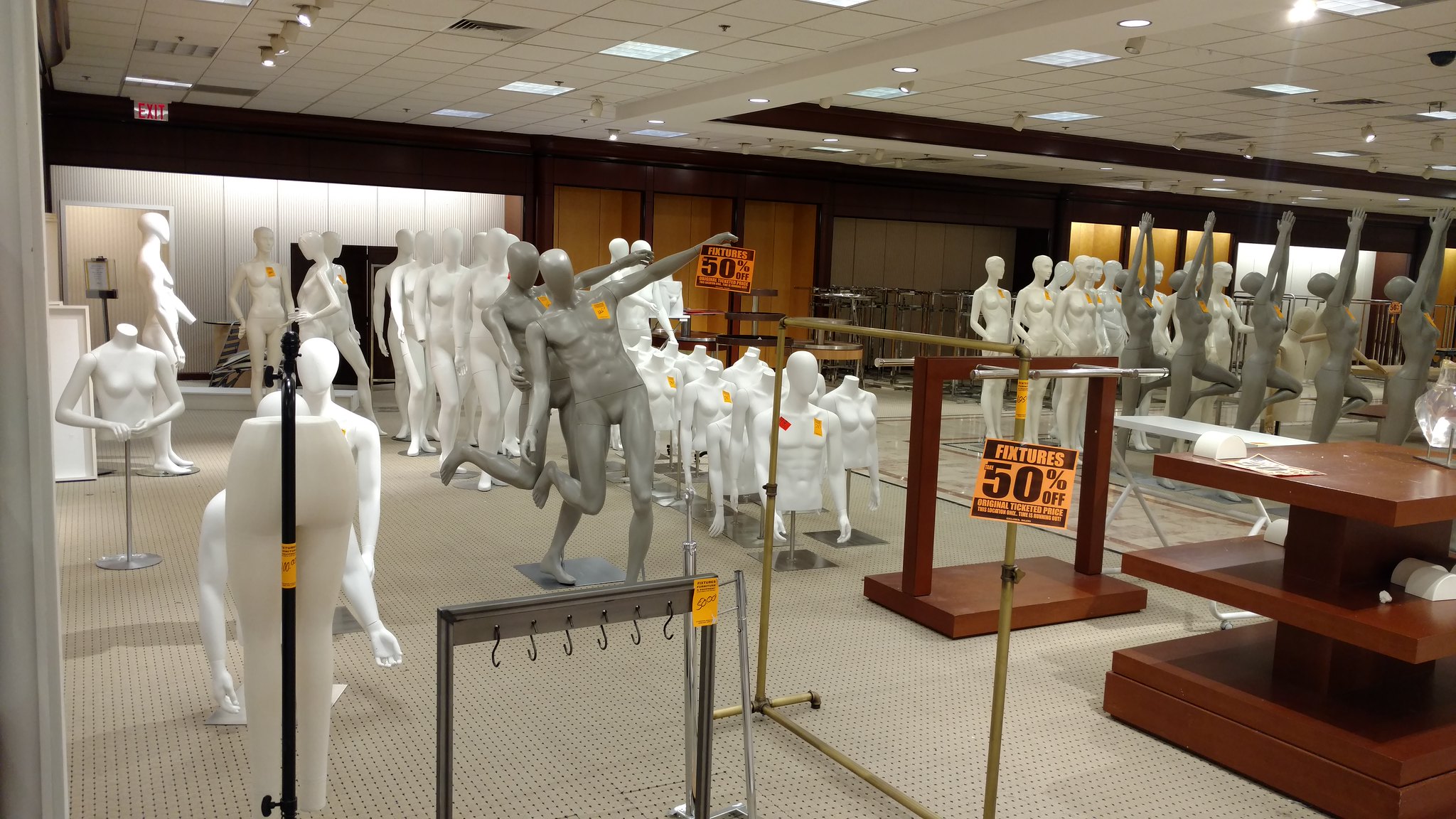The image showcases a spacious retail store characterized by a variety of lighting fixtures, including spotlights, track lighting, recessed lights, and halogen lamps behind ceiling tiles. The store's walls feature a mix of orange, yellow, gray, and a very light gray, almost white, specifically designed areas likely intended for merchandise display. The floor is a beige hue that complements the diverse color palette of the store.

Within this expansive room, numerous mannequins—both male and female—are positioned around the space. The mannequins are predominantly white and gray and are unclothed. Some of them are marked with orange and red tags, adding a splash of color amidst the neutral tones.

There are also several empty shelving units, made from a reddish wood, scattered throughout the store. These shelves are either bare or contain minimal debris, indicating a state of transition or clearance. At the forefront, a prominent orange sign announces, "50% off fixtures," suggesting a significant sale or store closing.